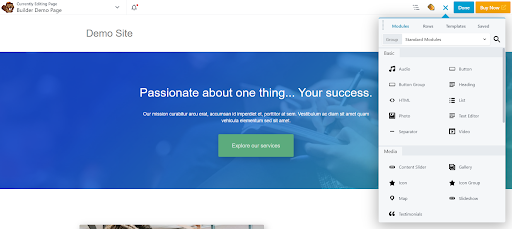This is a detailed and clean version of the caption for the website image described:

"The screenshot showcases a demo website, prominently marked with 'Demo Site' in the upper left corner alongside a small animal icon in brown. The header includes the phrase 'Demo Page.' On the right side, there is an orange 'Buy Now' button next to a blue box with white text that is too small to read entirely. Adjacent is a blue 'X' mark. Below the header, a visually appealing image features shades of blue blending into each other with the motivational phrase, 'Passionate about one thing, your success,' accompanied by smaller white text underneath. Further down, a green box labeled 'Explore Services' is visible. The main section depicts a close-up of a person writing in a book, showing only their hands. On the right side, a pop-up window with various icons and text, which is too small to decipher, appears above a search bar. Below the main blue-themed area is another partial image, with roughly an eighth of its content visible."